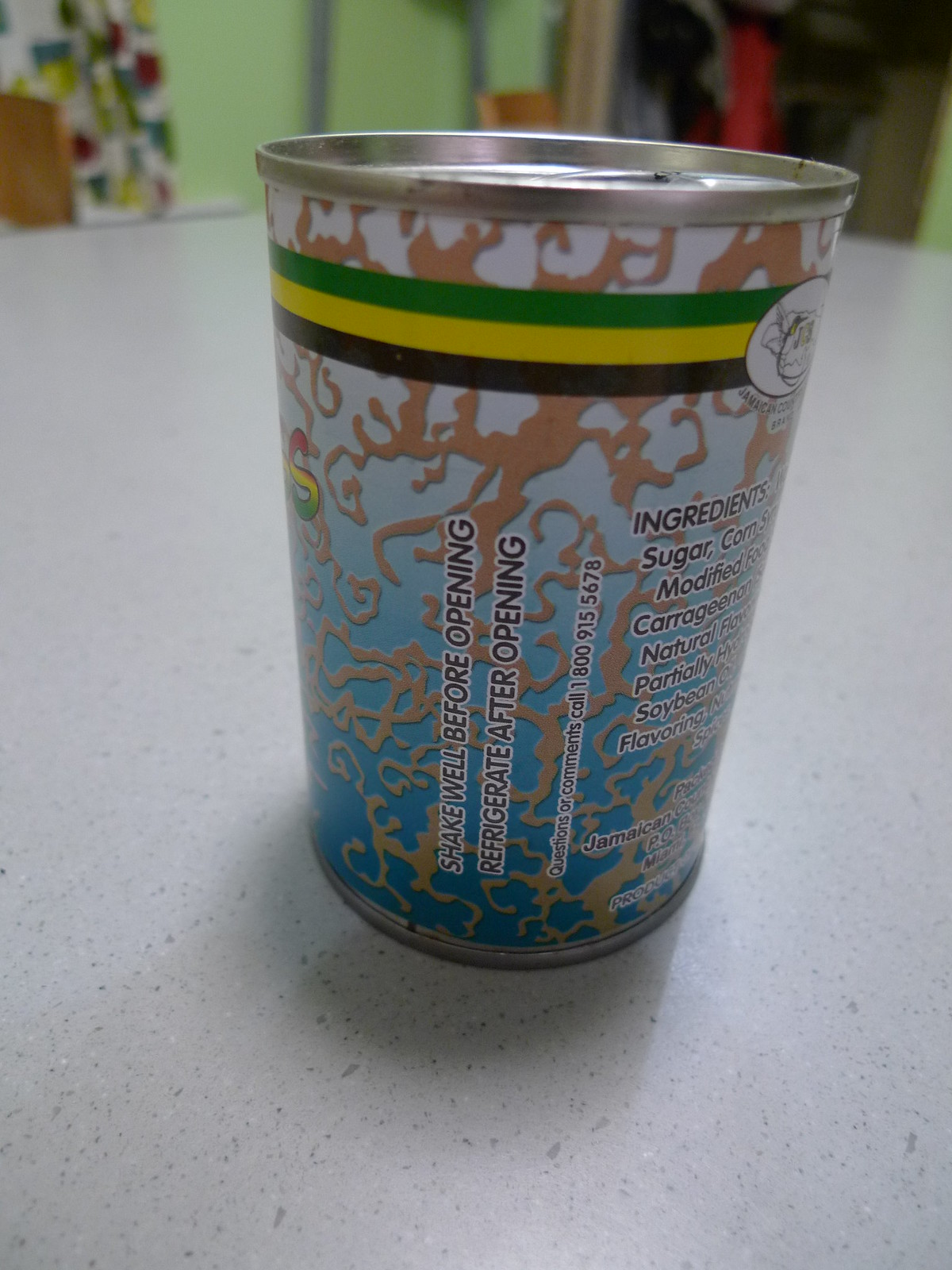This photograph captures a canned food item, housed within a metallic silver can that has a colorful and intricate label design. The label features a white background that gradually transitions to a soft blue hue, adorned with tan-colored, squiggly lines for visual interest. Encircling the top of the can, there is a decorative strip composed of green, yellow, and black colors. Written along the side of the can in dark, readable font are instructions that advise, "Shake well before opening" and "Refrigerate after opening." Additionally, there is a customer service contact number provided: "Questions or comments? Call 1-800-915-5678." A partial list of ingredients is also visible in the same dark font, indicating transparency about the contents within. The can itself is situated on a light gray surface, adding a neutral backdrop that highlights the vibrant label details.